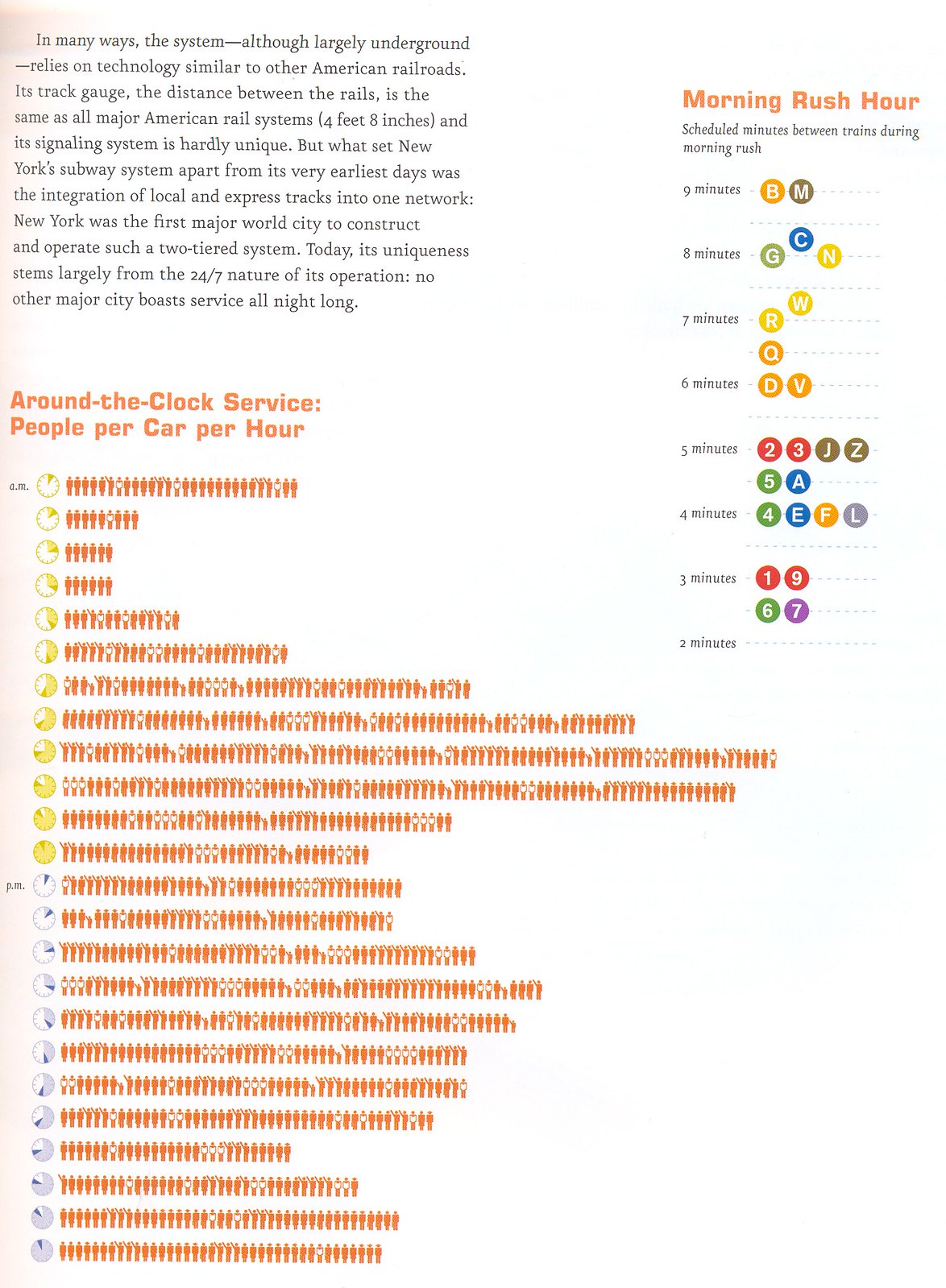This image presents a detailed study of the New York City subway system, emphasizing various operational and technological facets. Against a peach-hued, possibly faded background, the image combines a subway map with multiple charts and informational text. In the top left corner, a paragraph details the system's technological reliance, noting the standard American track gauge of 4 feet 8 inches and the integration of local and express tracks—a unique feature from its inception. The subway's 24/7 service is highlighted as a distinctive characteristic among major global cities.

On the right side of the image, a section labeled "Morning Rush Hour" outlines the schedule minutes between trains during this busy period. Listed beneath are intervals ranging from 2 to 9 minutes, accompanied by corresponding train lines such as the B, M, G, N, and others, along with numerical designations like 1, 2, 3, 4, 5, and more. Each interval shows specific trains assigned to it, with two minutes notably having no trains listed.

To the left, the chart displays data on "Around-The-Clock Service People Per Car Per Hour," represented by small figures indicating passenger density throughout the day. It shows peak occupancy during afternoon hours, with a noticeable decline as the evening progresses. Overall, the image is a comprehensive visual representation of the New York City subway's operational dynamics, from its technological underpinnings to its passenger flow during different times of the day.